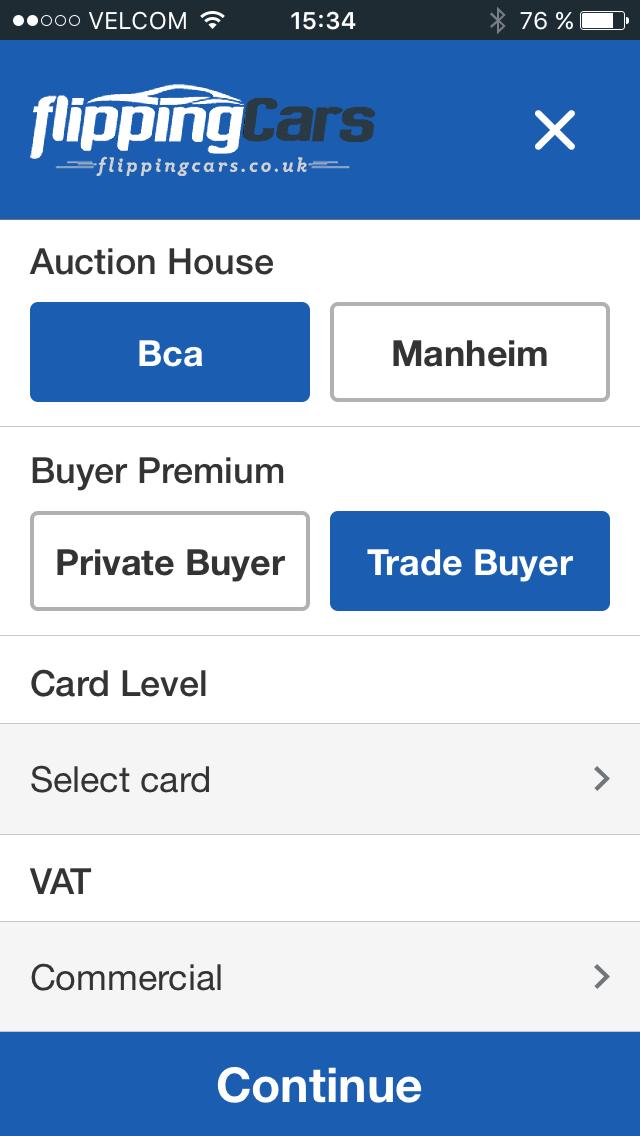The image is a colorful, detailed screenshot of a smartphone display, captured at 15:34 with the battery at 76%. The connectivity status shows Velcom service with two out of five bars, and Bluetooth is turned off, indicated by its faded gray icon. The primary focus of the screenshot is an app titled 'Flipping Cars,' where 'Flipping' appears in white text and 'Cars' in black over a blue banner background. The website linked to the app is flippingcars.co.uk, and the interface visible is a form related to auction houses.

On this form, the user can select between auction houses BCA and Mannheim, with BCA currently selected, highlighting it in blue. Under the "Buyer Premium" section, choices between 'Private Buyer' and 'Trade Buyer' are available, with 'Trade Buyer' selected. Further down, the user can select their card level via an option labeled 'Select Card,' accompanied by a dropdown arrow, though it appears no card has been chosen yet. The VAT section gives an option of 'Commercial,' which is selected by the user. At the bottom, there is a blue 'Continue' button with white text to proceed further.